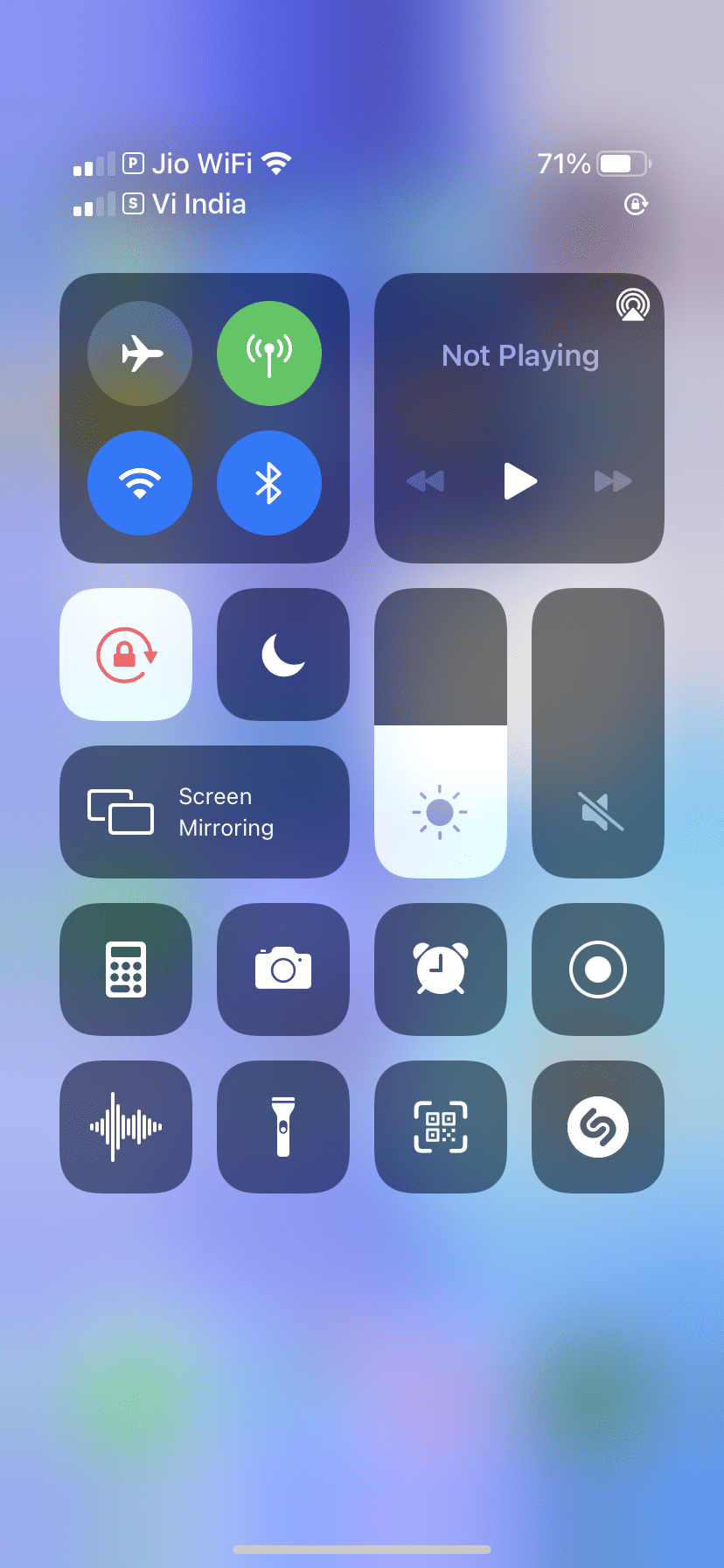This detailed image portrays a cell phone screen set in portrait orientation, showcasing an array of settings and icons. The background of the screen features a muted palette with variegated shades of purple, transitioning to green toward the bottom. 

Starting from the top of the display, clear white letters indicate the phone's network signal strength with "2 of 4 bars," adjacent to which is a white-outlined square with the letter "P." The text "Geo Wi-Fi" is displayed next to a full-strength Wi-Fi signal icon. Below this, another set of white letters indicates "2 of 4 bars" alongside an outlined square containing the letter "S," with the text "Vi India" accompanying it.

On the top right corner, "71%" is displayed next to a horizontal battery icon depicting the current charge level. Directly beneath it, a small circle containing a lock and an arrow encircling it is depicted. 

Moving down, two dark squares are aligned horizontally. The left square features four distinct icons in its quarters: a gray circle with a white airplane icon (presumably for airplane mode), a green circle with a white signal strength icon, a blue circle with a white Wi-Fi signal icon, and another blue circle with the Bluetooth symbol. The right square indicates media control settings with the text "Not Playing" and displays a play button flanked by fast-forward and rewind arrows in light gray.

Below these squares are additional icons. The top row includes a white square with a red lock and arrow, and a dark square with a half-moon icon (possibly for do not disturb mode). Adjacent to these is a rectangle labeled "Screen Mirroring" with two superimposed screen outlines, and to its right, a brightness adjuster with a sun icon at the bottom.

Continuing right, another rectangle houses the mute indicator at its bottom. Below this row, four square icons represent various functions: a calculator, a camera, an alarm clock, and a circle with a button inside, possibly for Google Assistant or a similar service.

The final row features four more icons from left to right: an indetermined waveform, a flashlight, an icon with four squares at its center within an outline, and a white circle with two interlocking Cs, likely denoting logo-related functionality.

This comprehensive arrangement of symbols provides clear quick-access to various phone settings and functionalities adorned on a visually distinct background.